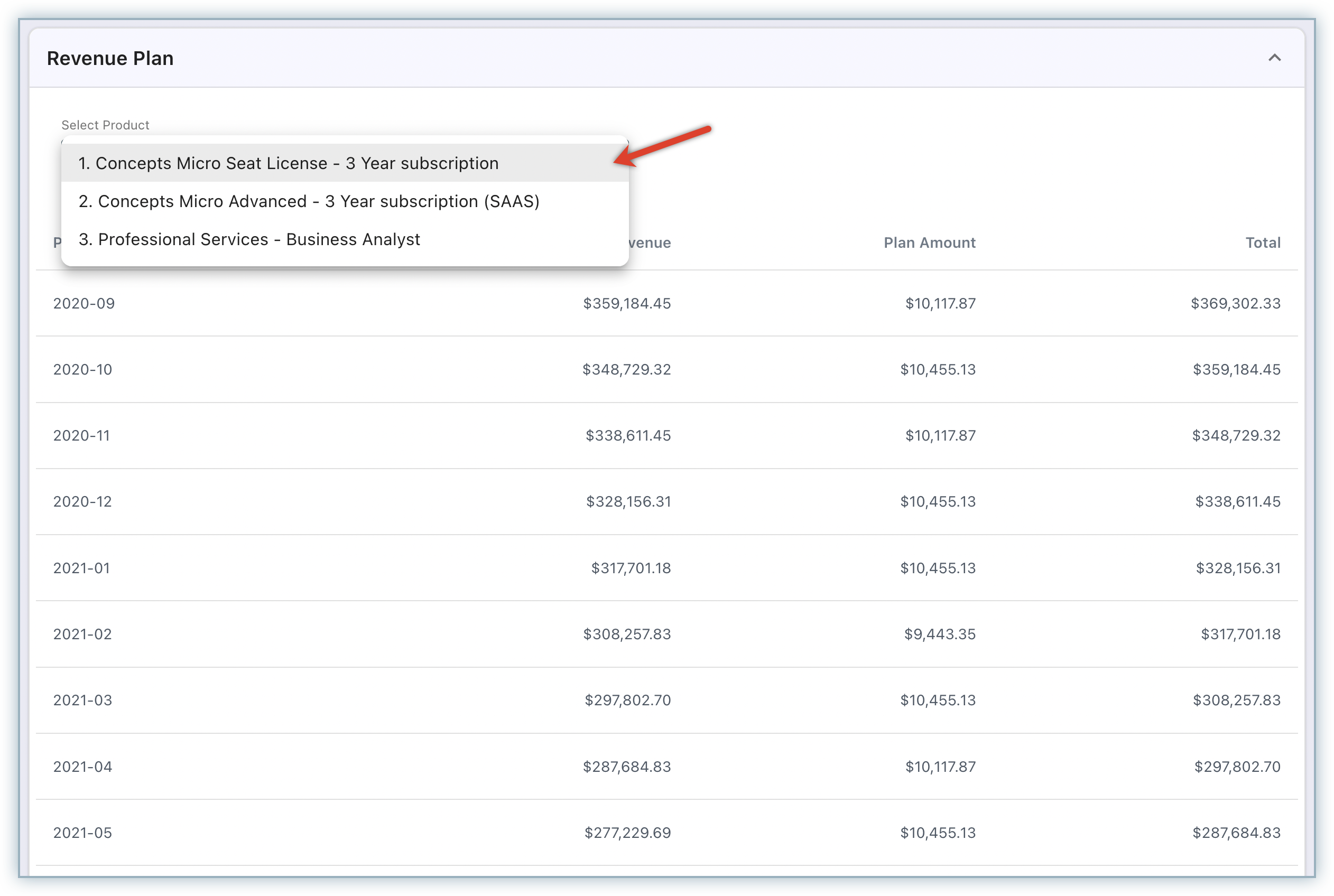### Detailed Descriptive Caption

This image is a screenshot of an application or software interface, likely related to revenue planning. The screenshot features a square layout with a thin blue-gray outline and a subtle blurred shadow along the outer edges, giving it a slight 3D effect.

#### Top Section:
At the very top of the image, there is a light gray bar. In the top left corner of this bar, bold black text in title case reads "Revenue Plan." Below this title, a thin gray border separates the header from the main content of the application.

#### Main Section:
The main section of the interface has a white background. At the top, there is a label that reads "Select Product" followed by an open drop-down menu. The first item in this drop-down list is highlighted in gray, indicating user selection or hover. The highlighted item reads, "1. Concepts Micro Seat License - 3-Year Subscription," with a red arrow pointing at it to possibly emphasize its importance. Below this, the second item in the drop-down list reads, "2. Concepts Micro Advanced - 3-Year Subscription (SaaS) 3 Professional Services - Business Analyst."

#### Data Table:
Behind the drop-down menu, there is a data table with approximately 10 to 12 rows of information. The drop-down menu partially obscures the table headers, but the following details can be discerned:

- **First Column**: Contains dates formatted as YYYY-MM. Examples include "2020-09," "2020-10," and "2020-11."
- **Second Column**: Labeled "Revenue," as inferred from partially visible text, although it's partially blocked by the drop-down menu. The first visible revenue amount is "$259,184.45," followed by similar amounts in subsequent rows.
- **Third Column**: Labeled "Plan Amount," displaying different plan amount prices. The first entry is "$10,117.87," followed by similar figures in the subsequent rows.
- **Fourth Column**: Labeled "Total," which appears to be the sum of the values in the "Revenue" and "Plan Amount" columns. The first entry in this column is "$369,302.33," which correctly sums the values from the first and second columns' corresponding rows.

This layout provides a detailed breakdown of revenue plans and associated financial details, although some information is obscured by the open drop-down menu.